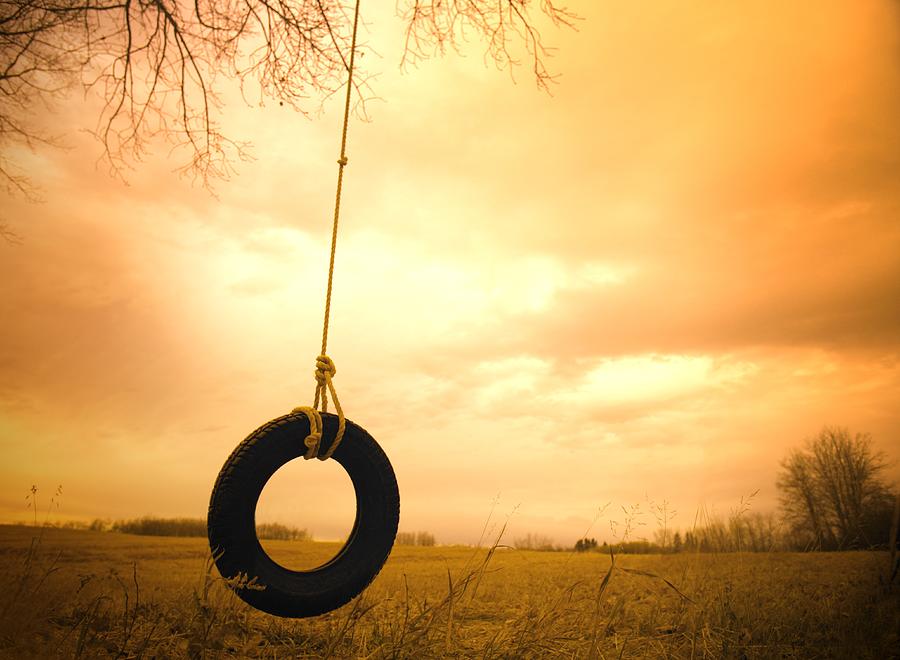This high-quality photograph captures a serene tire swing hanging from a tree, set against a vividly warm backdrop of an orange and yellow sky. The tire swing, made from a black tire and suspended by a yellow rope, is positioned slightly to the left of the image, with the rope descending from the top left corner where the tree's branches are visibly supporting it. The foreground is speckled with wild weeds, while the lower one-fifth of the image features a golden-hued grassy meadow. In the distance, a forest spans the horizon, its low-growing trees creating a soft silhouette against the sky. The overall tone of the image is golden and sepia-like, evoking an older, timeless quality reminiscent of dusk or a clouded sky filled with the diffused glow of the setting sun. This scene captures an empty, expansive field void of any human-made structures, emphasizing the solitary and peaceful ambiance.